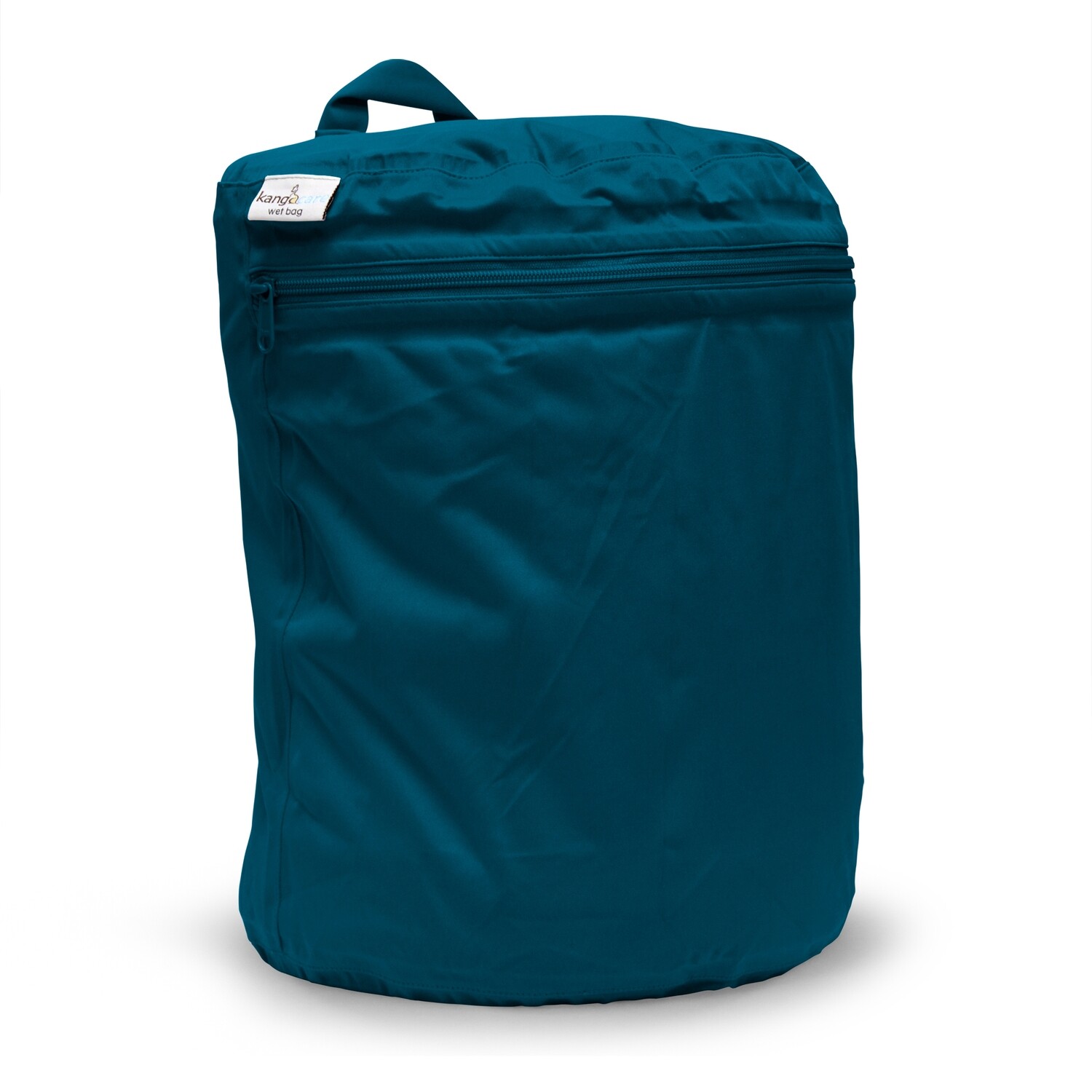The image features a tall, rectangular-shaped bag in a dark teal, almost sapphire-like color. The bag occupies the entire frame, set against a completely white background, lending a clean, minimalist aesthetic typical of a product sales photo. The bag has a fabric handle at the top, matching its dark teal hue. Beneath the handle, a turquoise zipper runs horizontally from one side to the other, blending seamlessly with the bag's fabric. A white tag with black text reading "kangaroo wet bag" is affixed near the top left corner of the bag, suggesting it is designed to either hold wet items or protect contents from moisture, ideal for outdoor activities or travel. A soft shadow beneath the bag adds a touch of depth to the otherwise stark white setting.